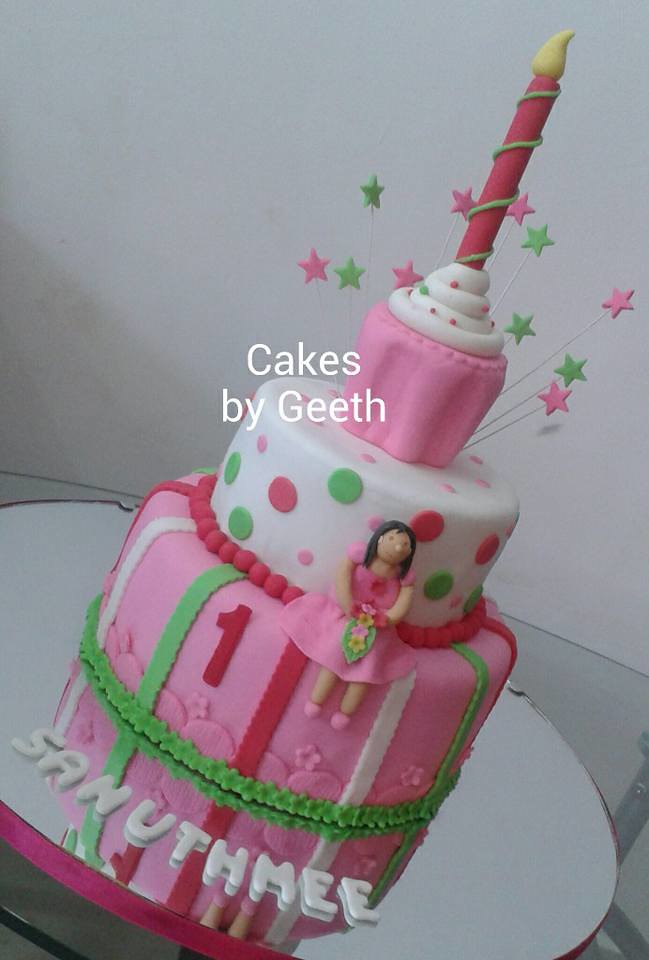The image showcases a stunning and professionally crafted, three-tiered birthday cake, beautifully decorated in shades of pink, red, green, and white. The bottom two tiers resemble classic cake tiers adorned with intricate patterns of stripes, polka dots, and green frosting ribbons, while the top tier creatively mimics a cupcake with white swirling frosting crowned by an edible candle. The bottom tier features the number "1," indicating the cake is for a first birthday celebration. 

Sitting on the bottom tier is an adorable figure of a little girl with long black hair, dressed in a pink dress and shoes, holding a floral wreath. This charming figure adds to the cake's overall cute and girly appeal without being overly so. The name "Sanuthmee" is elegantly written in icing beneath the cake, which sits upon a mirror, reflecting the ornate details. Central within the image is a watermark titled "Cakes by Geeth," showcasing the cake creator's name in white text. Each element, from the frosting dots to the edible decorations, highlights the artistry and professional craftsmanship that went into making this extraordinary celebratory cake.